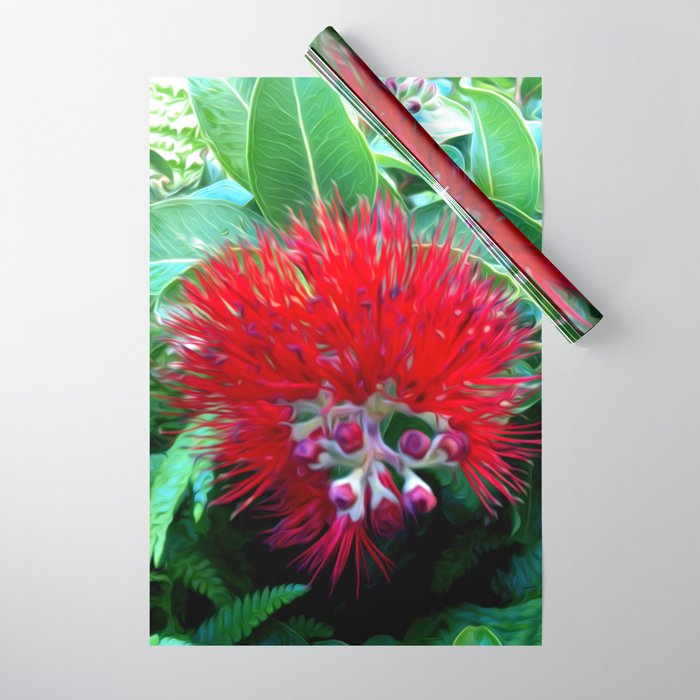This image features a highly detailed and vibrant illustration of a tropical flower. The flower boasts a vivid red, string-like structure at its top, resembling numerous threads with small white and purple buds interspersed throughout. Encircling the central stringy blossom are lush, high-definition green leaves that add to the richness of the scene. The flower appears to be depicted with a cluster of smaller, rose-like buds that have not yet bloomed, located near the center. Surrounding the primary floral illustration is a consistent gray background, suggesting the image might be lying on a table or wall. Additionally, there is a rolled-up piece of paper, potentially a poster, that sits on top of the illustration. This rolled-up paper seems to replicate the same floral design, integrating the red stringy material and green foliage, enhancing the layered complexity of the artwork.